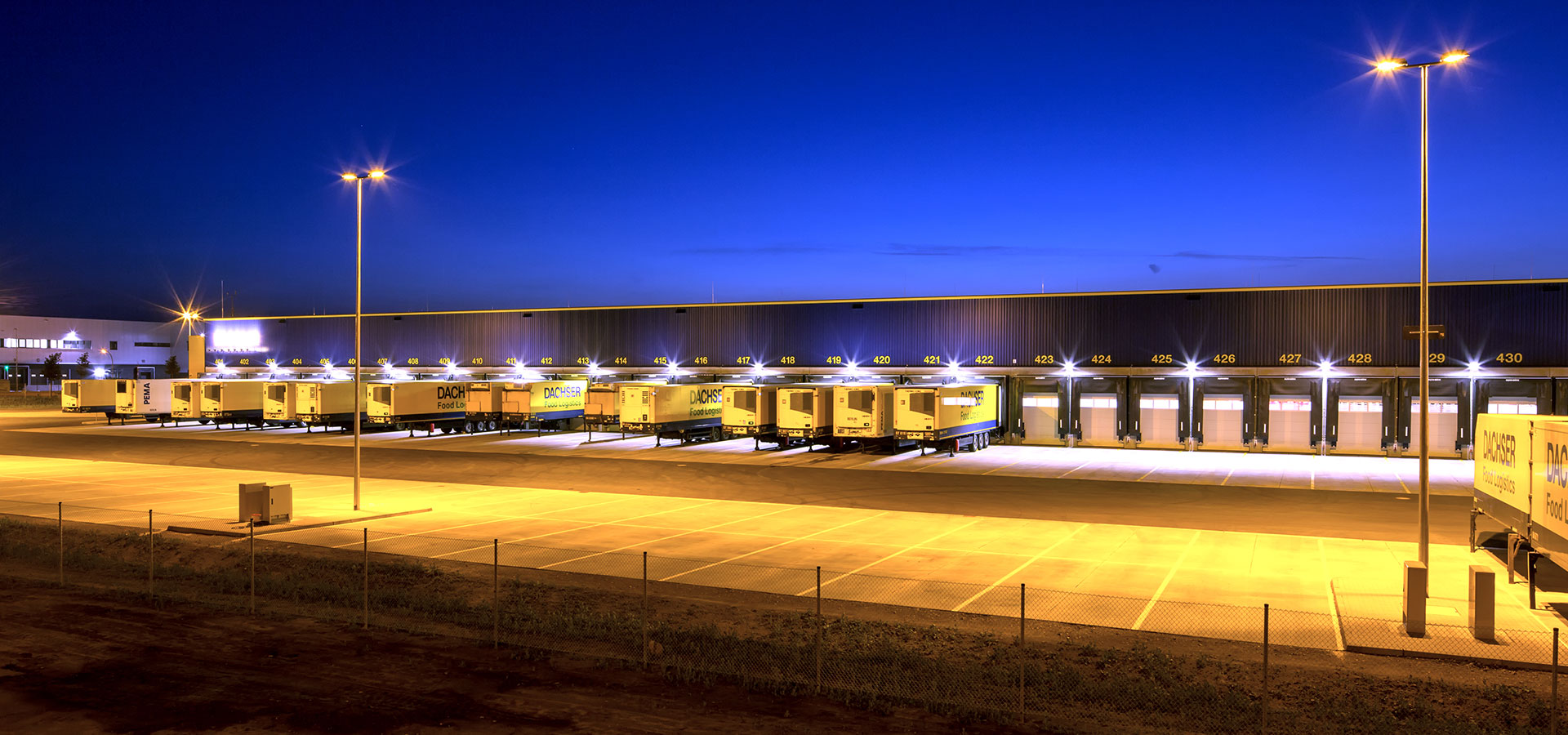The image is a photorealistic depiction of a large shipping depot or warehouse environment captured during dusk or early morning. The building, which appears to be used for industrial logistics, stretches from the right side towards the left but stops just short of the image's edge. Its exterior features black material near the top and numerous truck doors, each marked with a yellow number, designed for trucks to load or unload cargo.

In the foreground, a vast, paved parking lot with clearly marked yellow lines lies between the viewer and the building. Several light yellow trucks are backed into these open doors, ready for loading or unloading. Tall lampposts, emitting an orange glow, are located especially towards the bottom right and left sides of the image, illuminating the area. The sky is a deep, dark blue, indicating a time either at dusk or very early morning, adding a serene yet industrial atmosphere to the photograph.